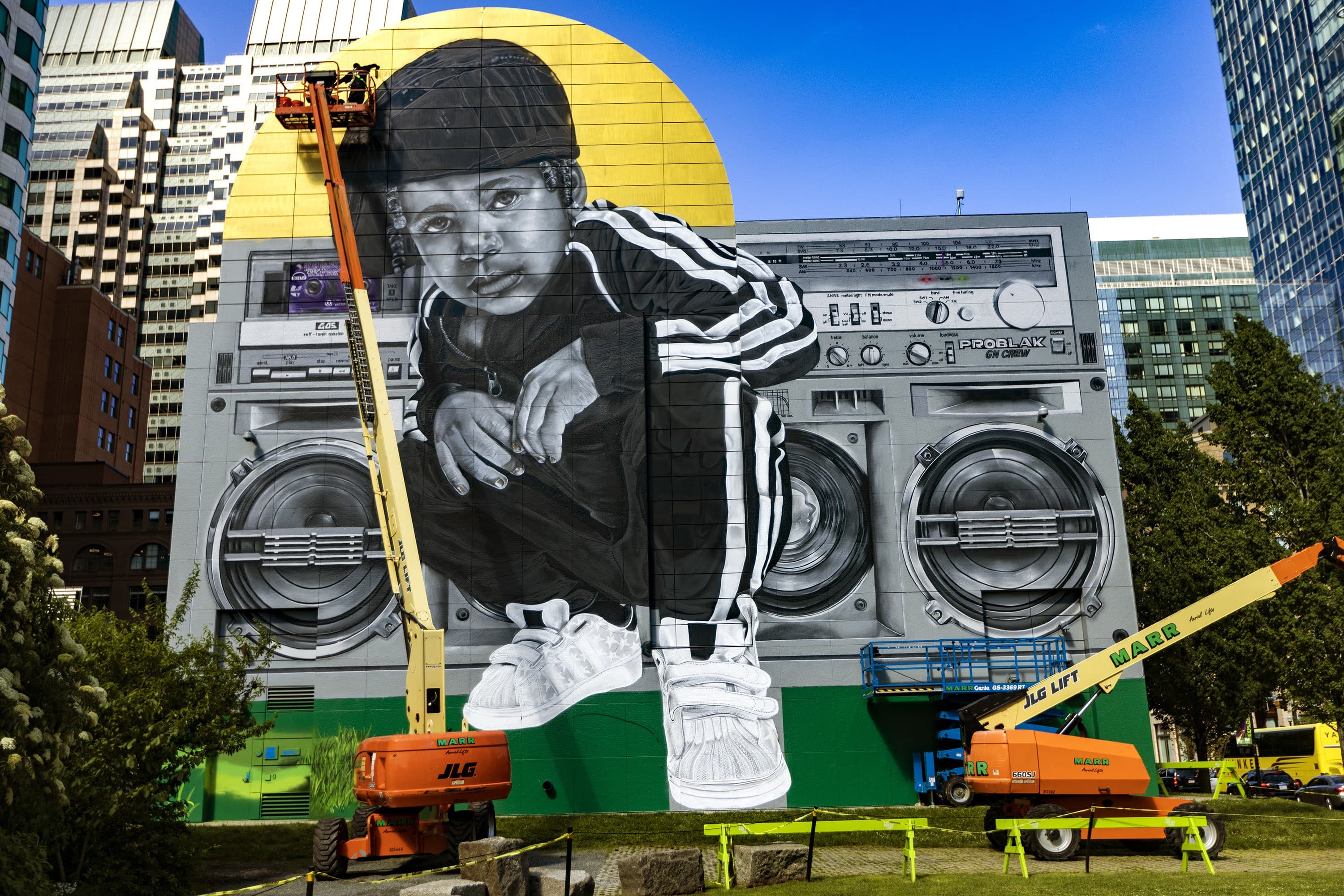This photograph captures an expansive urban mural set against the side of a large building, depicting a young African American boy, around 10 years old, rendered primarily in shades of black and white. The boy, who has a somber expression, sits on his heels facing the viewer. He is outfitted in a black tracksuit with striking white stripes running down the sleeves and legs, along with matching white high-top sneakers popular in the 1980s, and a black cap. Behind him looms a giant, light gray, 1980s-style boom box, enhancing the mural’s nostalgic vibe.

The boy appears to be seated on a green floor, with a touch of greenery visible beside his feet. Above him, a yellow circle resembling the sun fades into the background. The mural's surroundings feature tall apartment or office buildings, creating a dense cityscape. In the foreground, construction equipment painted in bright orange and yellow, resembling toy cranes, adds to the urban feel. The mural's setting includes a city square with patches of grass and bushes, adding a hint of nature amidst the urban sprawl.